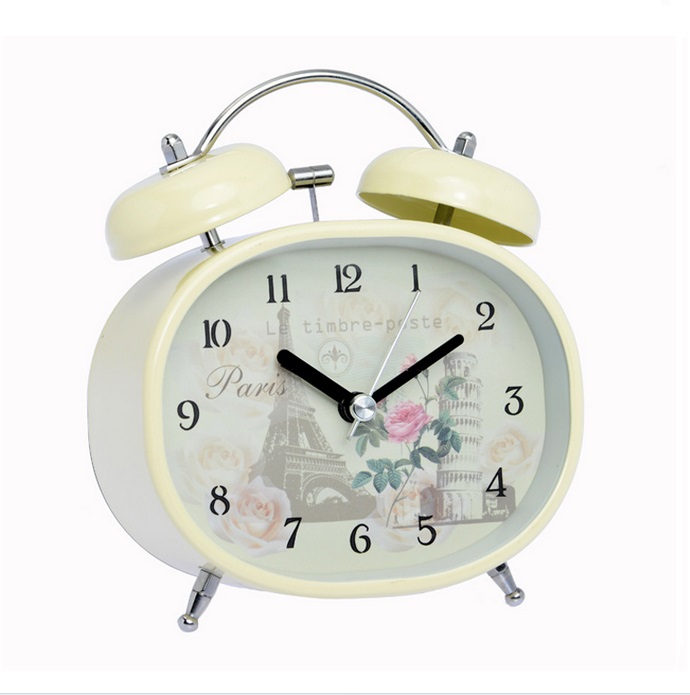This photograph showcases a vintage-style alarm clock, designed to evoke nostalgia with its classic aesthetic. Positioned against a pristine white background and placed on a matching white surface, the clock is likely a product image intended for an online store display. The clock itself is made of white plastic, featuring twin bells on top, also in white, with a silver handle bridging them. The base is white plastic, fitted with two small metal feet for support. 

The clock face is protected by a clear plastic cover and adorned with illustrations of iconic European landmarks, including the Leaning Tower of Pisa and the Eiffel Tower. The word "Paris" is prominently displayed in black font, adding to its thematic design. The clock’s numbers, 1 through 12, are also in black, ensuring clear legibility. The time is indicated by three hands—hour and minute hands in black, and a silver second hand—providing functionality wrapped in a charmingly retro presentation.